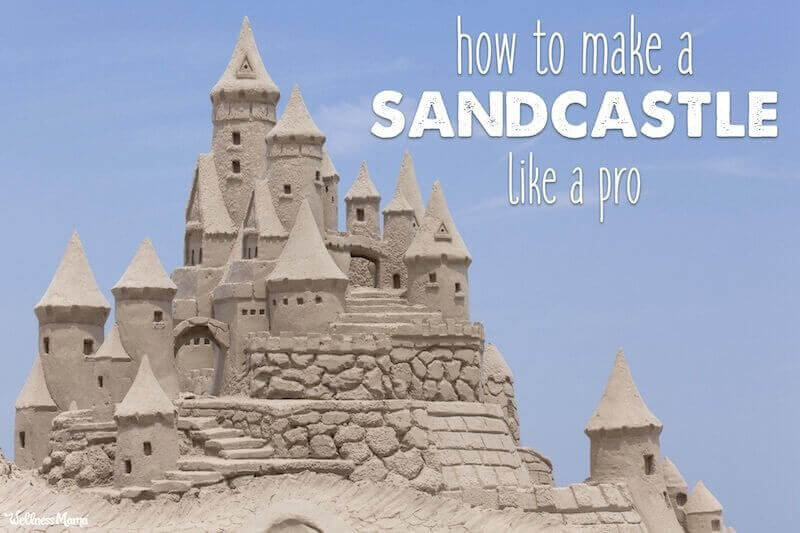The image features an intricate sandcastle set against a clear blue sky, suggesting the picture was taken during the day. The sandcastle is elaborate, with multiple levels and detailed designs. It includes a base layer adorned with sharp tower peaks and spiral-like spires, connected by arch bridges and staircases leading to higher sections. One prominent tower stands out with two rows of windows, unlike the other towers which typically have just one. The top right corner of the image contains the text "How to Make a Sandcastle Like a Pro" with "Sandcastle" in bold, white capital letters. In the bottom left corner, there is a watermark that reads "Wellness Mama."